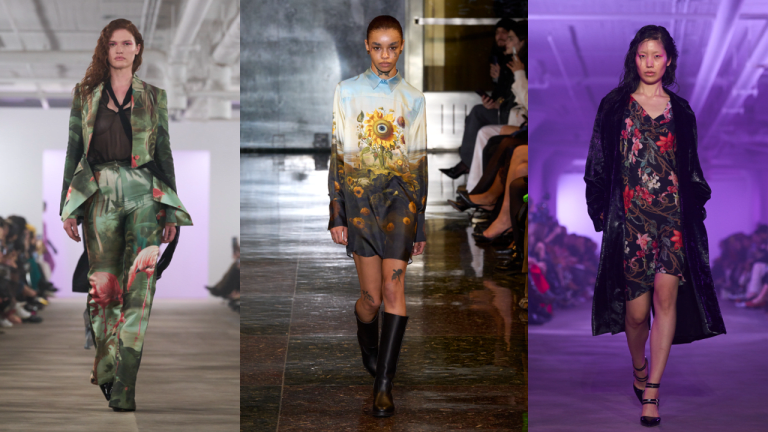The image is an amalgamation of three distinct color photographs, each featuring a different female model showcasing unique fashion styles. The photos are aligned side-by-side in portrait orientation, creating an expansive landscape image.

The first model on the left is dressed in a green camo-style outfit comprised of a printed blazer and matching pants with pink flamingo accents. She pairs this ensemble with a dark scarf tied around her neck and a black blouse underneath. She has long brown hair and walks on a beige runway, the wooden floor slightly visible, with a white projector backdrop and a white ceiling above her.

In the center, a young girl, approximately 13 years old, is styled in a short-sleeved shift dress that finishes at her thighs. The dress is adorned with a prominent sunflower graphic in the middle and is complemented by tall black leather boots. Her look is completed with dark makeup smudges and visible tattoos on her upper thighs, set against a background of a gray panel. She has short brown hair, and faint details of spectators are discernible along the edges.

The last model, an Asian young woman, graces the rightmost photograph in a black floral dress accented with red flowers, topped with an open black trench coat. She is styled in black high heels with ankle straps and carries an aura of sophistication as she walks along a cement floor, beneath a ceiling bathed in purple light. The purple background and hints of spectators on either side underline the vibrant setting. Overall, the cohesive integration of these fashion-forward images embodies the essence of contemporary runway photography.